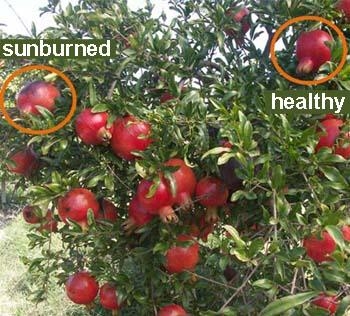This color photograph captures a partial close-up view of a pomegranate tree or bush laden with numerous deep red pomegranates. The tree's bright green leaves fill the entire foreground, providing a lush backdrop to the many round fruits, which somewhat resemble apples but feature a distinctive crown at the bottom. In the image, two pomegranates are specifically highlighted with orange circles and white pixelated text. On the top left, the circled pomegranate is labeled "sunburned," displaying a noticeable blackened top. On the top right, another circled pomegranate is labeled "healthy," indicating its pristine condition. At the bottom left corner, grass is visible beneath the tree. The photograph is devoid of people, animals, buildings, or any man-made structures, focusing solely on the natural elements.